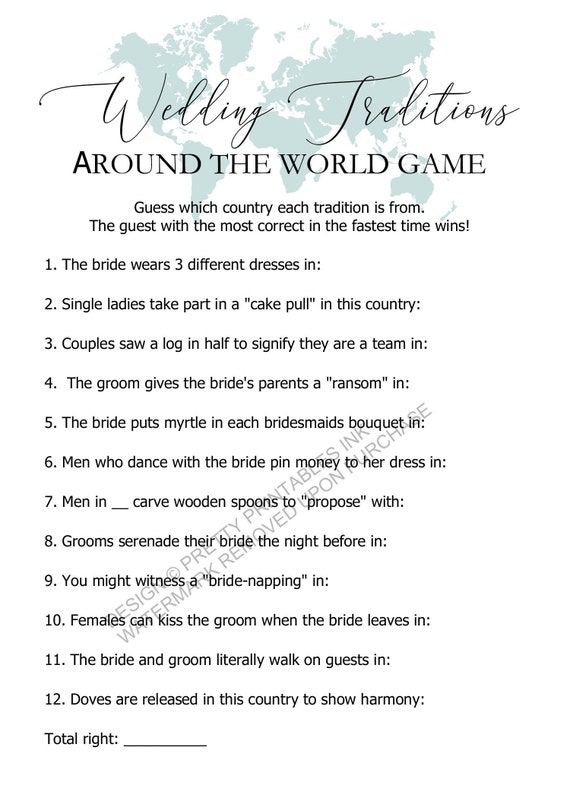This image depicts a detailed wedding game titled "Wedding Traditions Around the World." At the top of the page, there is a mint-green map of the world with the phrase "Wedding Traditions" elegantly written in cursive over it. Underneath, in bold lettering, it says "Around the World Game." The game challenges participants to guess the country each wedding tradition originates from, with points awarded for the most correct answers in the fastest time. The instructions are clearly printed beneath the title. There are 12 questions listed, each describing a unique wedding custom, such as "The bride wears three different dresses in..." or "Doves are released in this country to show harmony." A transparent black watermark, stating "design, copyright, pretty printables, ink, watermark removed upon purchase," overlays the image, marking it as a purchasable printable document possibly from an online source like Etsy. The page features a total score section at the bottom where participants can tally their correct answers.